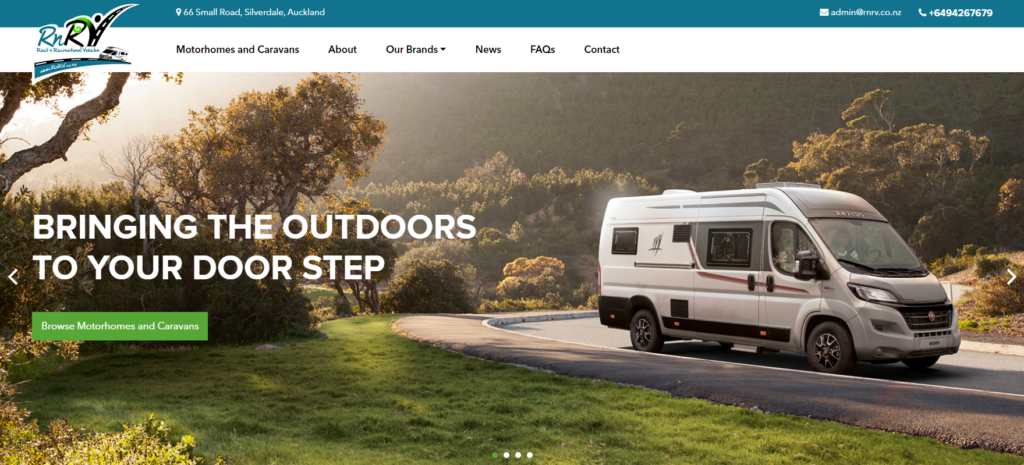In this screenshot, the top section features a blue banner displaying the text "66 Small Road, Silverdale, Auckland," along with contact information positioned on the upper right. The details read: "admin@rnrv.co.nz" and phone number "649-426-7679." Below the blue banner, a white navigation bar is visible on the left side, listing menu options such as "RNRV," "Motorhomes and Caravans," "About," "Our Brands," "News," "FAQs," and "Contact."

The main body of the screenshot showcases a vibrant, outdoor photograph taken in daylight, depicting a camper-style van traveling on a scenic mountain road. The white van with brown stripes is surrounded by lush, dark green trees, indicative of a summer or warm climate, as evidenced by the verdant grass and foliage. Superimposed text to the left of the van reads, "Bringing the outdoors to your doorstep" in large, bold white letters. Below the text, a green box offers a call to action: "Browse Motorhomes and Caravans."